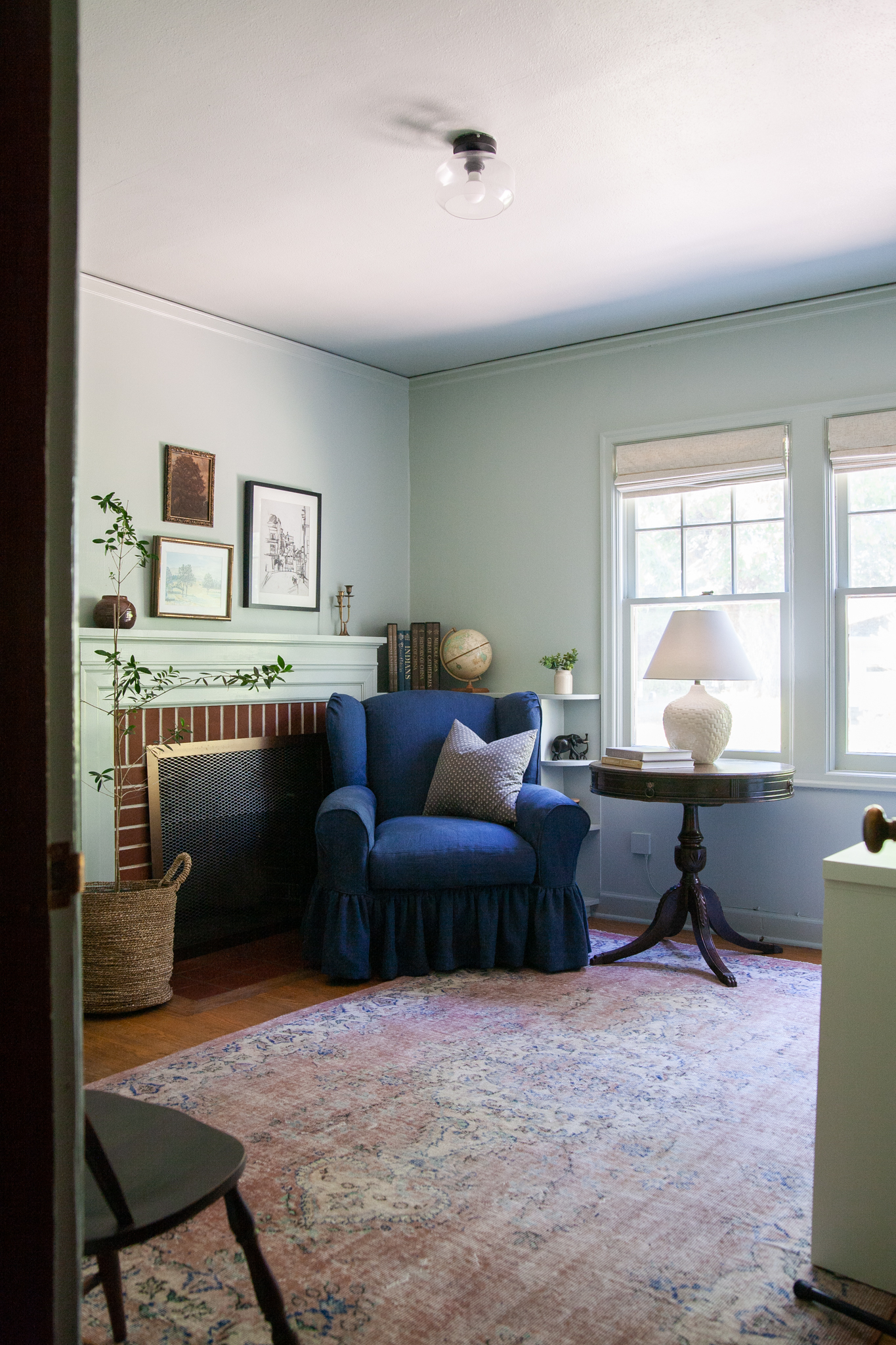This image captures a cozy, well-decorated living room scene. Dominating the foreground is a worn and faded red carpet adorned with intricate patterns, over which rests an assortment of furniture. On the left side, near the doorway through which we view the room, is a chair. A blue recliner with a single pillow sits prominently in the middle of the room, positioned close to a fireplace that features a distinctive gold grate. To the left of the fireplace is a woven basket holding a plant, adding a touch of greenery. Above the fireplace, three frames featuring architectural artwork are neatly arranged. 

Adjacent to the recliner, on its right, stands a traditional brown round side table topped with a white lamp. Behind this table is a bookcase or shelf that holds several books and a globe. Additional details include a white dresser or bookcase on the far right and two windows that allow natural light to brighten the space. The color palette of the room includes rich shades of blue, brick red, gold, white, gray, black, and tan, creating a warm and inviting atmosphere.